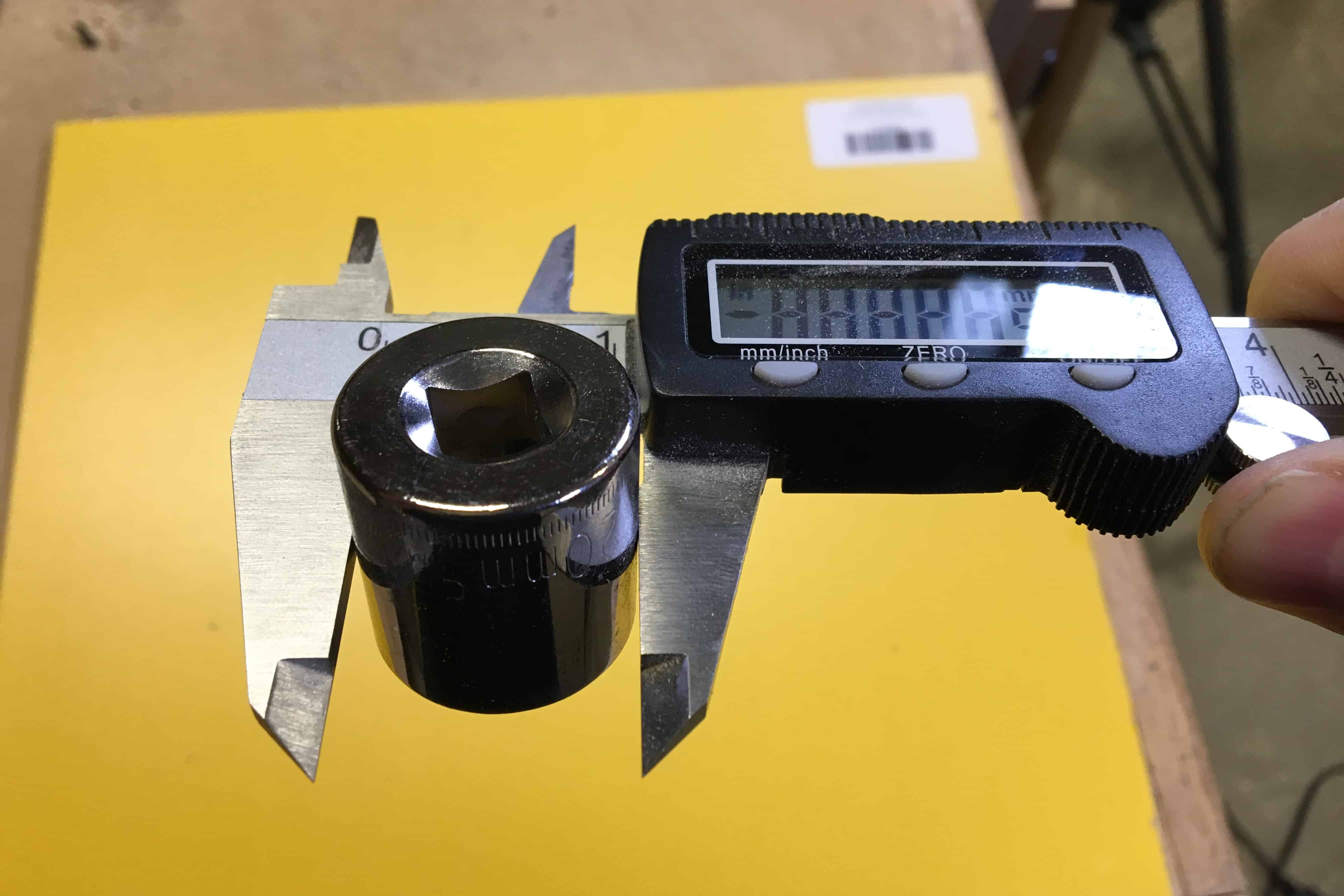This close-up photograph captures a digital caliper used for precise measurement, possibly of a cylindrical object. The device itself is black plastic and features a small monitor displaying numeric readings readable as four followed by a one, which might indicate a measurement. Below the screen are buttons marked "mm/inch" and "zero," while another button isn't fully visible due to glare. The caliper's jaws secure a black cylindrical object, and it is held steadily by a light-skinned person with slightly dirty fingernails. In the background, the yellow surface of a manila folder with a white UPC label partially covers a light brown wooden table. Bits of a chair and some concrete floor are also visible.